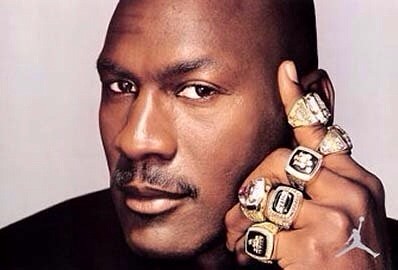In this digital photo, Michael Jordan, the legendary African-American basketball player, is the central focus against a whitish cream background. He is looking directly at the camera, but his eyes are subtly directed towards the right, giving the impression that he is glancing out of the corner of his eyes. Jordan, recognizable by his bald head and thin eyebrows, wears a black shirt. His facial hair includes a thin mustache.

His left hand, adorned with multiple gold rings that feature black centers and gold inscriptions, rests against the right side of his face from the viewer's perspective. The detailed arrangement includes two rings on his index finger, one on his middle finger, two on his ring finger, and one on his pinky finger. In the bottom right corner, the iconic Air Jordan Jumpman logo, depicting him leaping with legs spread and holding a basketball, adds a distinctive touch to the image.